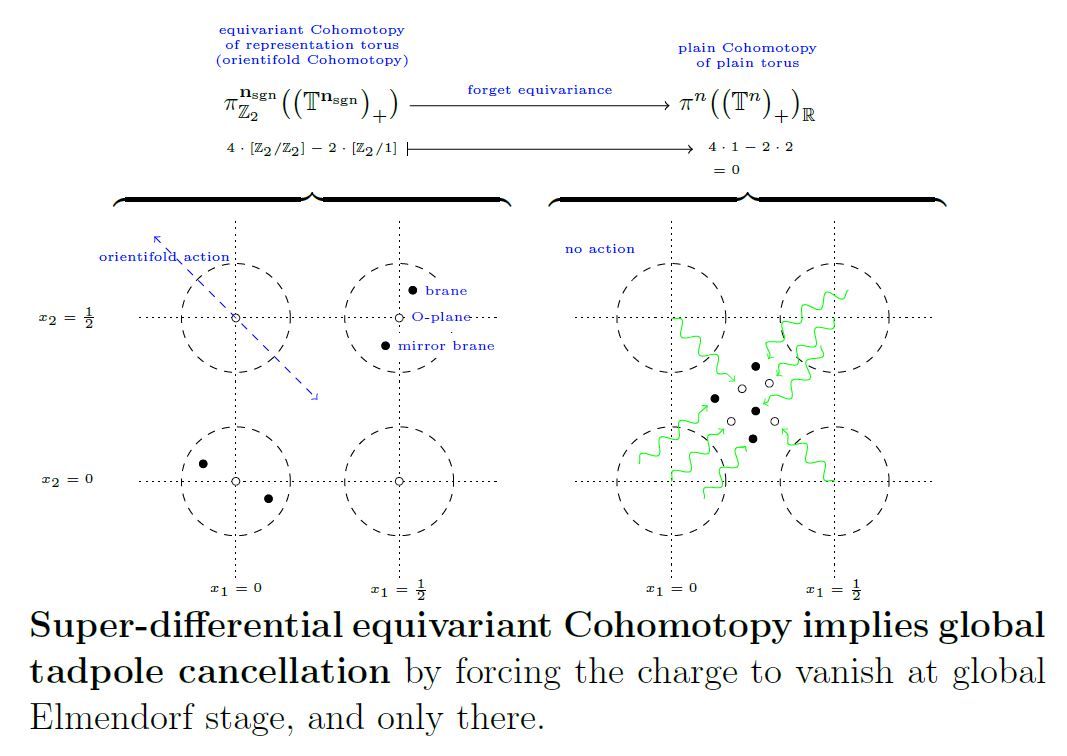The image is a complex diagram filled with mathematical symbols, numbers, and various annotations. At the bottom, there is a black text caption that reads, "Superdifferential Equivariant Cohomotopy Implies Global Tadpole Cancellation by Forcing the Charge to Vanish at Global Elmendorf Stage and Only There." Near the top, annotations in blue and black include "Equivariant Cohomotopy of Representation Taurus (Orient Fold Cohomotopy)," and "Forget Equivariance, Plane Cohomotopy of Plane Taurus.”

The diagram features two main sections resembling tic-tac-toe grids, each with two horizontal and two vertical lines intersecting, creating small circular nodes at each intersection. On the left side, there are sequences of equations in blue text connected by blue arrows, labeled "Orient Fold Action." On the right side, similar sequences feature green arrows with the label "No Action." The left section also includes horizontal brackets enveloping dashed circles grouped in fours on either side.

The top portion continues with equations and variables in both blue and black text. Overall, the image presents an intricate mix of equations, diagrams, and textual elements, set against a white background, illustrating advanced theoretical concepts in mathematics and physics.